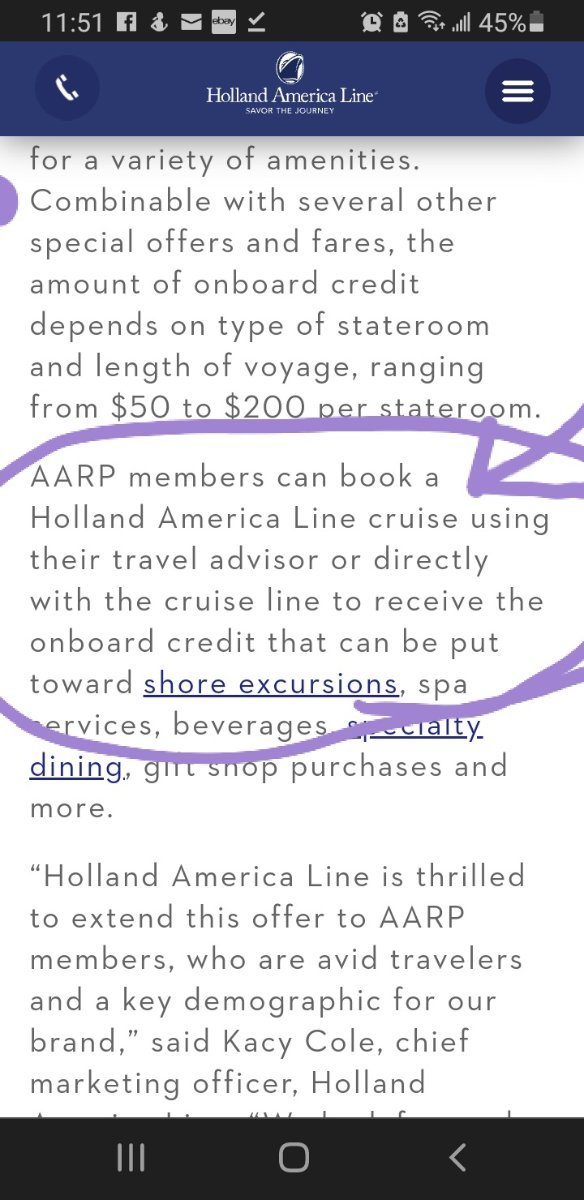**Descriptive Caption:**
The screenshot displays the home screen of a smartphone with several elements arranged across the top and middle of the screen.

- **Top Black Strip:**
  - On the left side, the time "11:51" is shown, followed by a series of icons: a Facebook icon, an email icon, and an eBay icon. There is also a check mark over a line.
  - Towards the center to the right, there are icons for an alarm, a recycle symbol, signal bars indicating data or Wi-Fi strength, and a battery indicator showing "45%".

- **Middle Blue Band:**
  - On the left side, there is a phone icon.
  - In the center, the text reads "Holland America Line - Savor the Journey."
  - On the right side, there are three horizontal lines stacked on top of each other, suggesting a menu.

Below this blue band, additional promotional details about a Holland America Line cruise are provided:

- The text highlights various anemones, amenities, and offers available for AARP members. It mentions that the amount of onboard credit depends on the type of stateroom and length of the voyage, ranging from $50 to $200 per stateroom.
- The promotion details are emphasized with a purple circle and arrow, indicating that AARP members can book a Holland America cruise through a travel advisor or directly with the cruise line to receive the onboard credit.
- This onboard credit can be used for various purposes, such as shore excursions, spa services, beverages, specialty dining (partially obscured by the purple arrow), gift shop purchases, and more.

The promotional content concludes with a statement in blue and underlined text, indicating that AARP members can book to receive these benefits. Following this, there is a message from Holland America Lines expressing their enthusiasm to extend this offer to AARP members, who are identified as avid travelers and a key demographic for the brand.